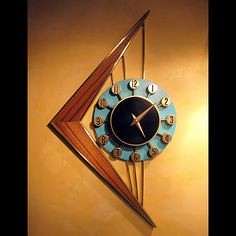In this image, we see an extremely small circular clock positioned centrally within a distinctive composition. To the left of the clock, there is a brown, boomerang-shaped object, resembling a bow, emphasizing an artistic element. Extending from this boomerang shape are three brown strings, vertically aligned from top to bottom, which articulate a connection to the clock at the center.

The clock itself is light blue, featuring numbers that are arranged within white circles. The numbering follows a traditional pattern: 12, 1, 2, and 3 are situated on the right-hand side; 4, 5, and 6 at the bottom; 7, 8, and 9 on the left-hand side; and 10, 11, leading back up to 12 at the top.

The clock's hands indicate a specific time: the minute hand is positioned between the numbers 1 and 2, while the hour hand points towards the number 5. The overall background features a blend of light brown and gold hues, adding a subtle depth to the image. On the very outer edges, both the left and right sides fade into a stark black background, framing the entire scene and drawing the viewer's focus towards the intricate details of the clock and its surrounding elements.